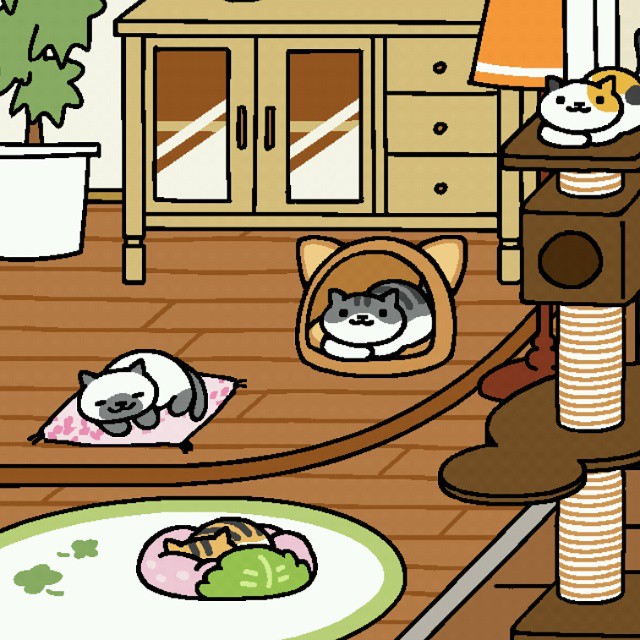This is a vibrant and detailed illustration from the mobile game Neko Atsume, where players attract cats to their homes with food. The indoor setting features a cozy, cartoon-style scene with bright colors and intricate details. Central to the image are four cats, each occupying different spots within the room. 

On the right, perched atop a multi-level brown cat tree, is a calico cat lounging comfortably with a content expression. In the foreground, a white rug with a green border and green flower design hosts two more felines: an orange and black striped tabby cat is peacefully sleeping on a pink cushion, while nearby, a gold and gray striped cat snoozes inside a pink and green cat bed. 

Adding to the cozy atmosphere, a brown enclosed cat bed shaped like a cat head with ears sits adjacent to the rug, harboring a striped gray and white tabby cat. The background reveals more homey details, including wood flooring, a beige credenza, and a potted plant, enhancing the inviting ambiance of this cat-filled sanctuary.